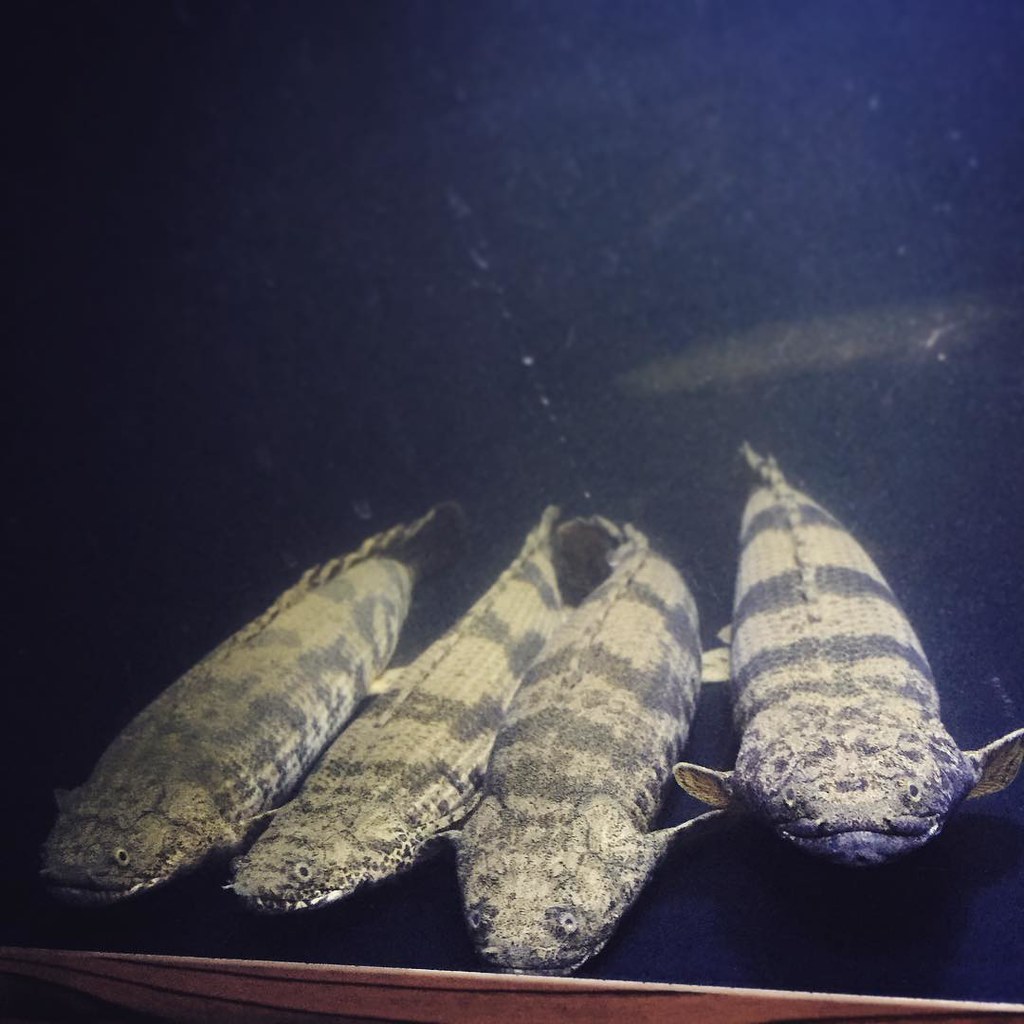The image captures a dimly lit aquarium with a blue interior and a brown frame at the bottom. Central to the scene are four distinct fish, each displaying a unique mix of grayish-white, brown, and black stripes. These fish, resembling amphibians or alligators with their elongated bodies and amphibian-like faces, are positioned horizontally at the bottom of the tank, almost appearing as if they are staring out through the glass. Their yellow eyes with black pupils add to their striking appearance. Additionally, there is a fifth fish, slightly blurred due to the water, swimming towards the left in the upper right corner of the image. The overall focus remains on the four side-by-side fish at the bottom, drawing attention to their unique and detailed features.